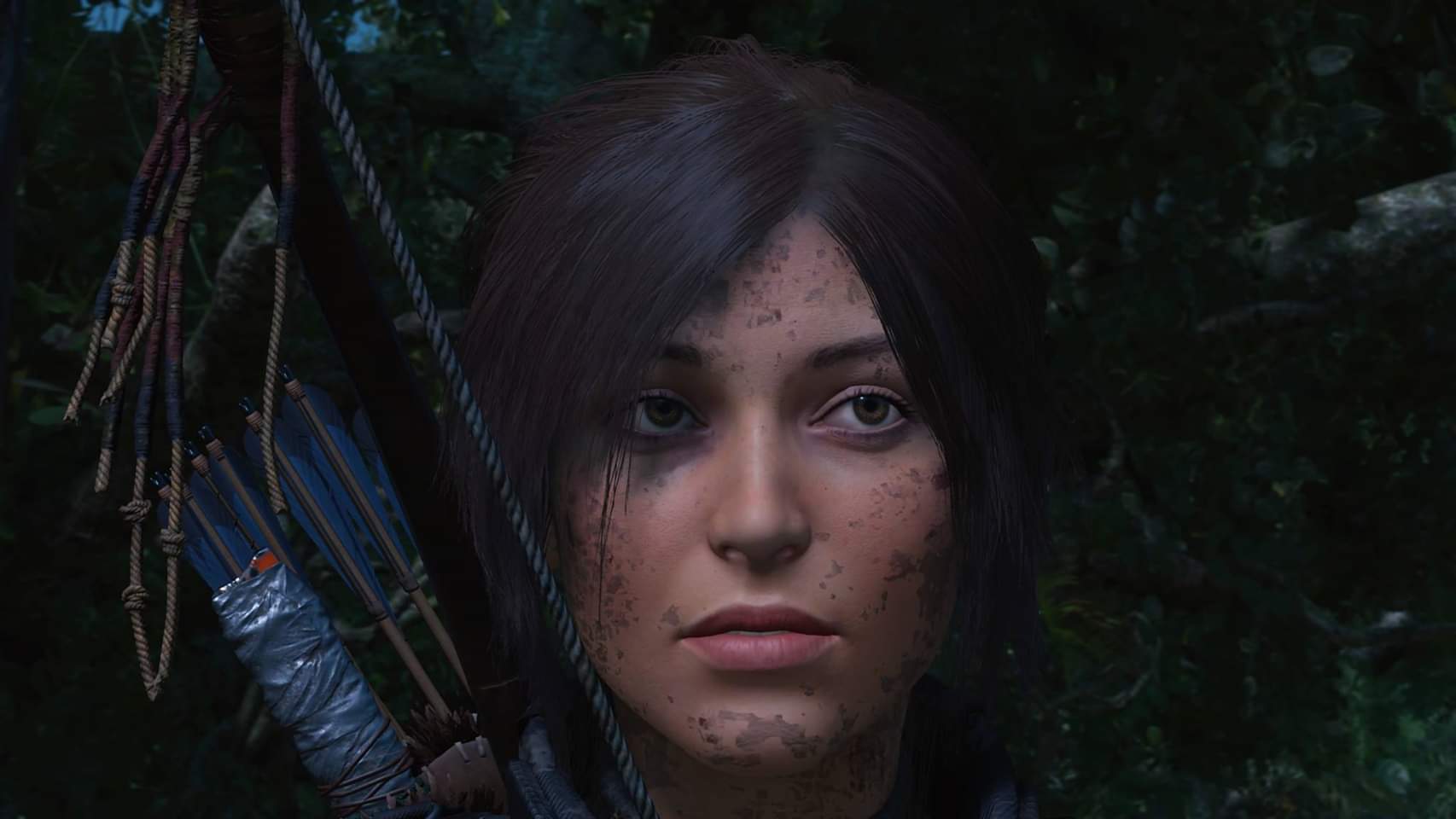In this striking, computer-generated image, a woman emerges from dense jungle vegetation, the vibrant greens of the thick foliage forming a vivid backdrop. Her face, neck, cheeks, chin, and forehead are splattered with mud, lending an aura of rugged determination. Her expressive hazel eyes are directed upwards, conveying a sense of focus and vigilance. Her brown hair is either pulled back or cropped short, adding to her fierce, warrior-like presence. On her back, she carries a bow and a quiver of arrows, the arrows made of wooden shafts with blue fletching. One cluster of arrows is wrapped in gray plastic, hinting at their use and preparation. The overall composition evokes a sense of survival and readiness in a wild, untamed environment.